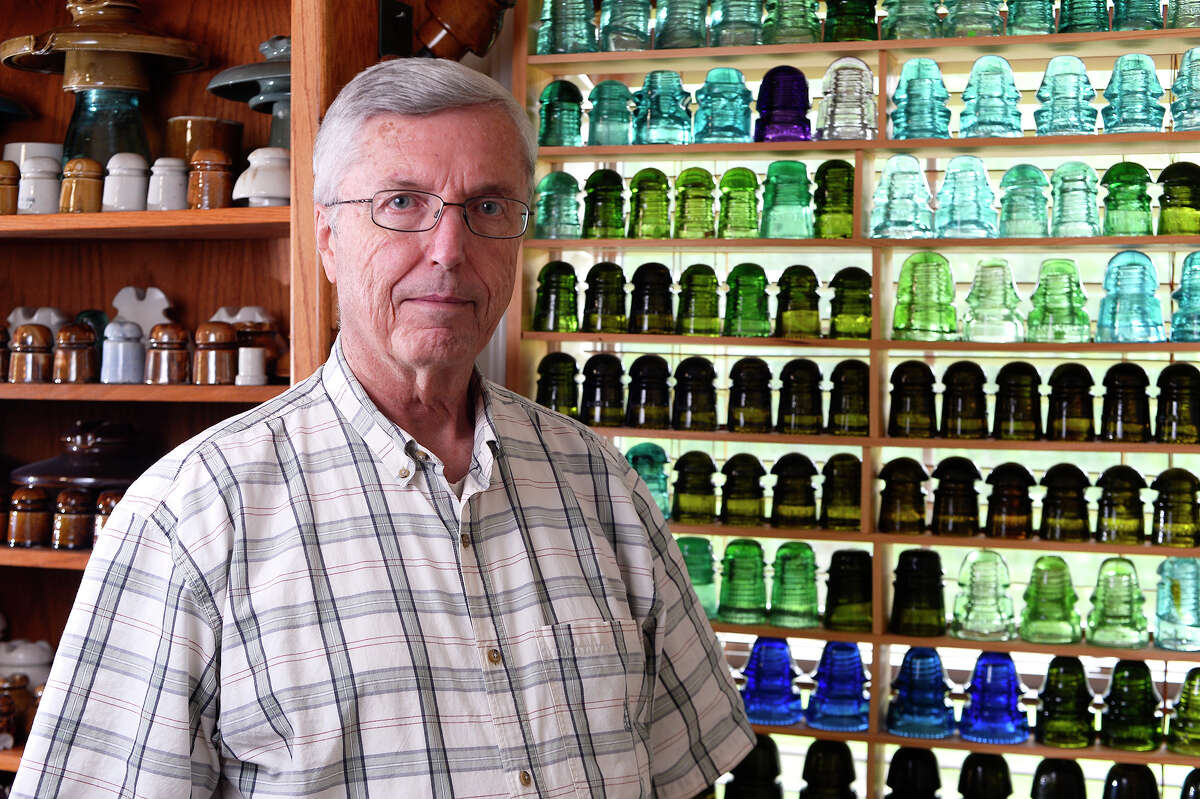An older Caucasian man with predominantly white hair, interspersed with some dark gray strands, stands at the forefront of the image. He wears rectangular-framed glasses and a white button-up shirt with blue plaid details. The man, who appears to be in his 70s or 80s, has blue eyes and a neutral expression, and he gazes directly at the photographer. In the background, there is an extensive collection of various glass and ceramic objects displayed on wooden shelving units.

The shelving on the left side of the man hosts a vibrant array of colorful glass jars that resemble sea glass buoys from the past. These jars—coming in shades of light blue, dark blue, dark green, and light green—are displayed on slightly misaligned wooden shelves, creating a whimsical and nostalgic atmosphere.

On the right-hand side, the display features more solid, ceramic-like items, primarily in hues of brown and white with some appearing to be porcelain. These objects, which may remind one of salt and pepper shakers, are also housed in a wooden shelving unit, but without the same visually striking backlighting as the glass jars on the left. This arrangement gives a subdued, rustic feel to that side of the image. The eclectic assortment of jars and shakers, combined with the man's AI-like appearance, lends the image a slightly surreal, yet compellingly detailed, quality.